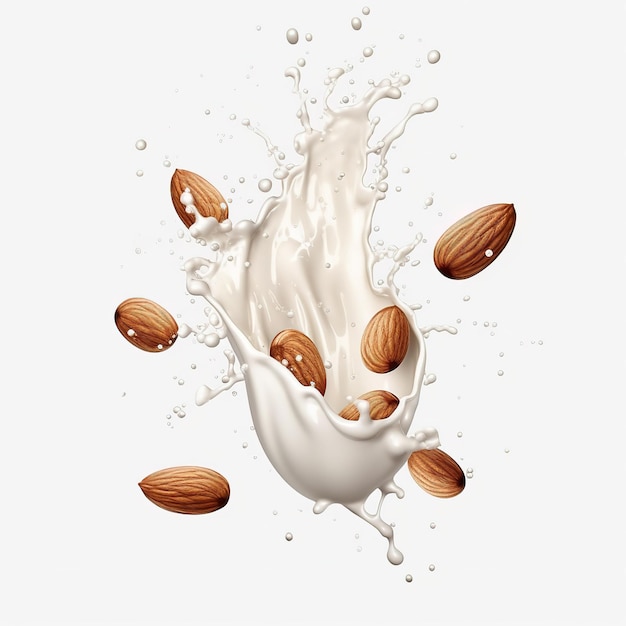This digital art image is a detailed illustration of almond milk in motion, capturing a dynamic scene where the milk is depicted in a mid-air splash forming a curved, bowl-like shape. The milk, which is entirely white and shiny, suggests a wet, liquid nature. Surrounding and interacting with this splash are eight brown almonds, with three almonds nestled inside the curved shape and five scattered around it. Tiny droplets of milk are visible, indicating motion and fluidity. The background is a light gray, providing a neutral backdrop that keeps the focus on the central elements. This evocative depiction possibly intended as a visual representation of almond milk, may serve as an advertisement, emphasizing the natural ingredients used.